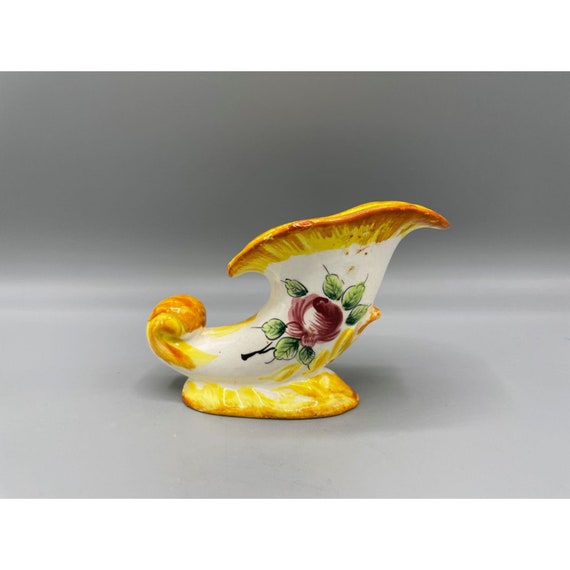This is a photograph of a ceramic, antique-style piece with an ambiguous design resembling both a cornucopia and a mushroom. The piece features a horn-like shape, widening at the top with a flared lip, and stands elegantly on a base. The top part is primarily amber and yellow, with varying shades creating a wave-like pattern towards the back. The midsection is white and adorned with a hand-painted, pinkish wine-colored rose surrounded by seven vividly green leaves. The intricate detailing suggests it could be used as a gravy boat, a vase, or simply as a decorative item. Possibly made from porcelain, its old-fashioned aesthetic hints at craftsmanship from a bygone era. The overall look, with its looping tail and rich colors, offers a unique combination of both functional and artistic appeal.